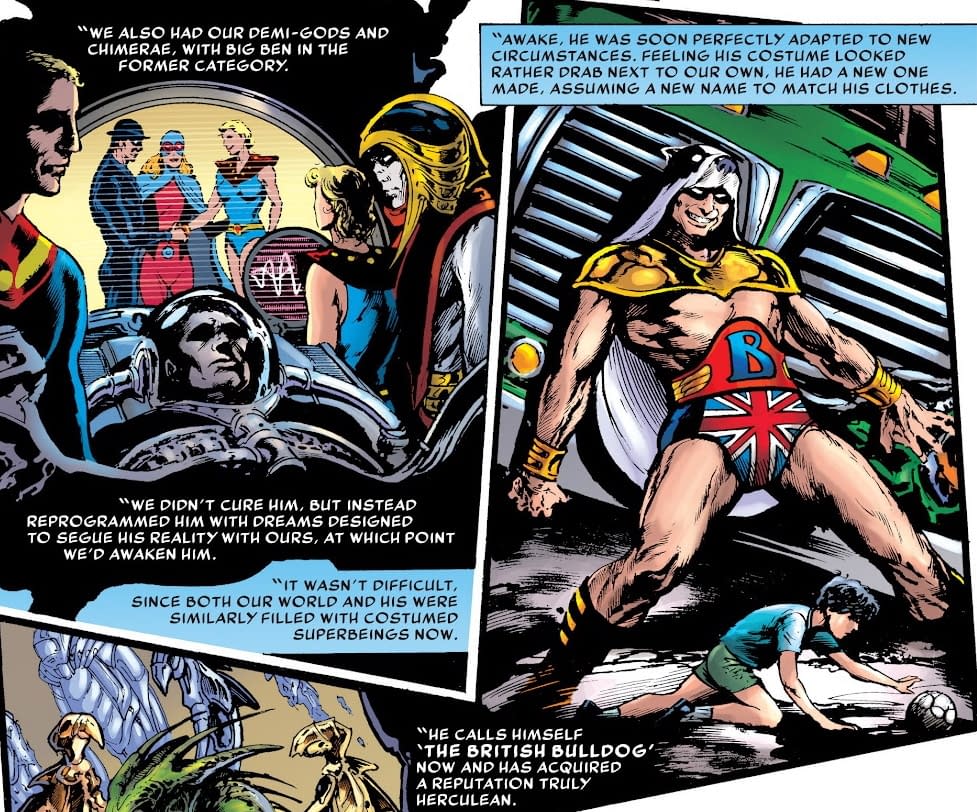In this image of a comic book strip, several detailed scenes are depicted. In the upper left corner, a character with short blonde hair, wearing a blue tight shirt with a red collar and a yellow stripe, reminiscent of a Superman-like figure, is highlighted in a white-text-on-black-background caption that reads, "We also had our demigods and Shimmeray with Big Ben in the former category." Nearby, a man in a spacesuit with a globe helmet is lying inside a mechanical object, resembling an operating table. Below this, another caption reads, "We didn't cure him, but instead reprogrammed him with dreams designed to seg his reality with ours, at which point we'd awaken him," and adds, "It wasn't difficult since both our world and his were similar, filled with costume super beings now."

On the far right, there is a striking character that looks like Thor, wearing British flag-themed tights, a red belt with the letter "B," and a gold-plated shoulder protector, resembling a WWE belt. This character, referred to as the British Bulldog, is muscular with a bare chest and legs and a panda helmet. He is seen heroically holding back a large green vehicle, potentially saving a crawling boy from being hit. Above this scene, a text box with black text on a blue background adds more context: "Awake, he was feeling adapted to new circumstances, feeling costume will drab next our own he had a new one made to match his clothing."

The artwork also hints at other fantastical elements, such as portals and aliens, suggesting a rich and intricate storyline filled with beings of extraordinary abilities.